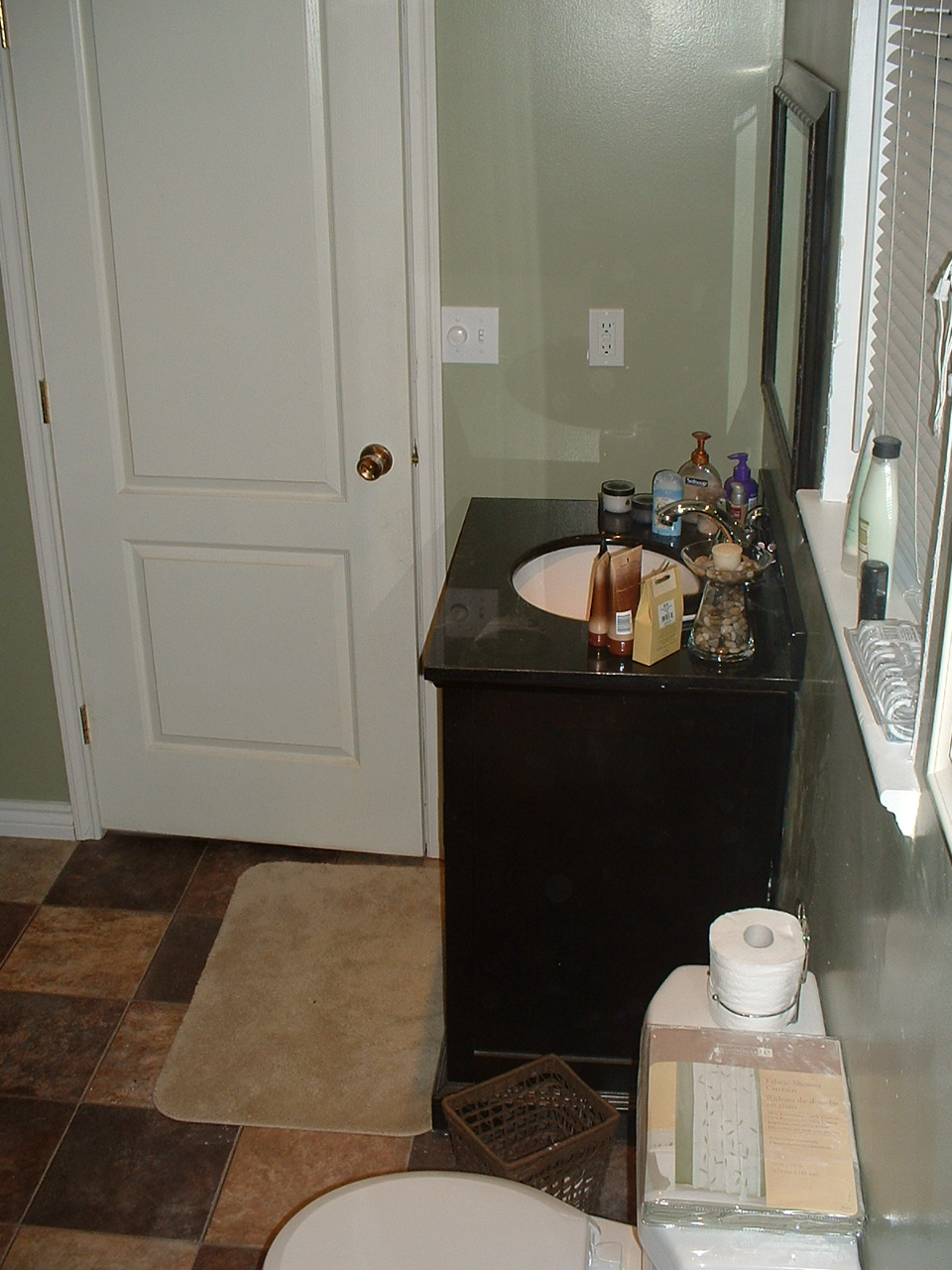A photograph taken from within a bathroom, capturing a view towards the mostly closed door. The door, which is slightly ajar, is aligned with an exhaust fan and a light dimmer switch. Several electrical outlets are also visible. In the foreground, a toilet with the bottom lid closed can be seen. A spare roll of toilet paper rests on the tank lid in a small receptacle. Adjacent to the toilet is a dark brown and tan checkered floor mat positioned next to a sleek black sink cabinet. The chrome faucet stands out against the dark sink, which is cluttered with various personal care products, including skin care items, hand soap, and fragrances. To the right of the sink, there is a wastebasket completing the scene.